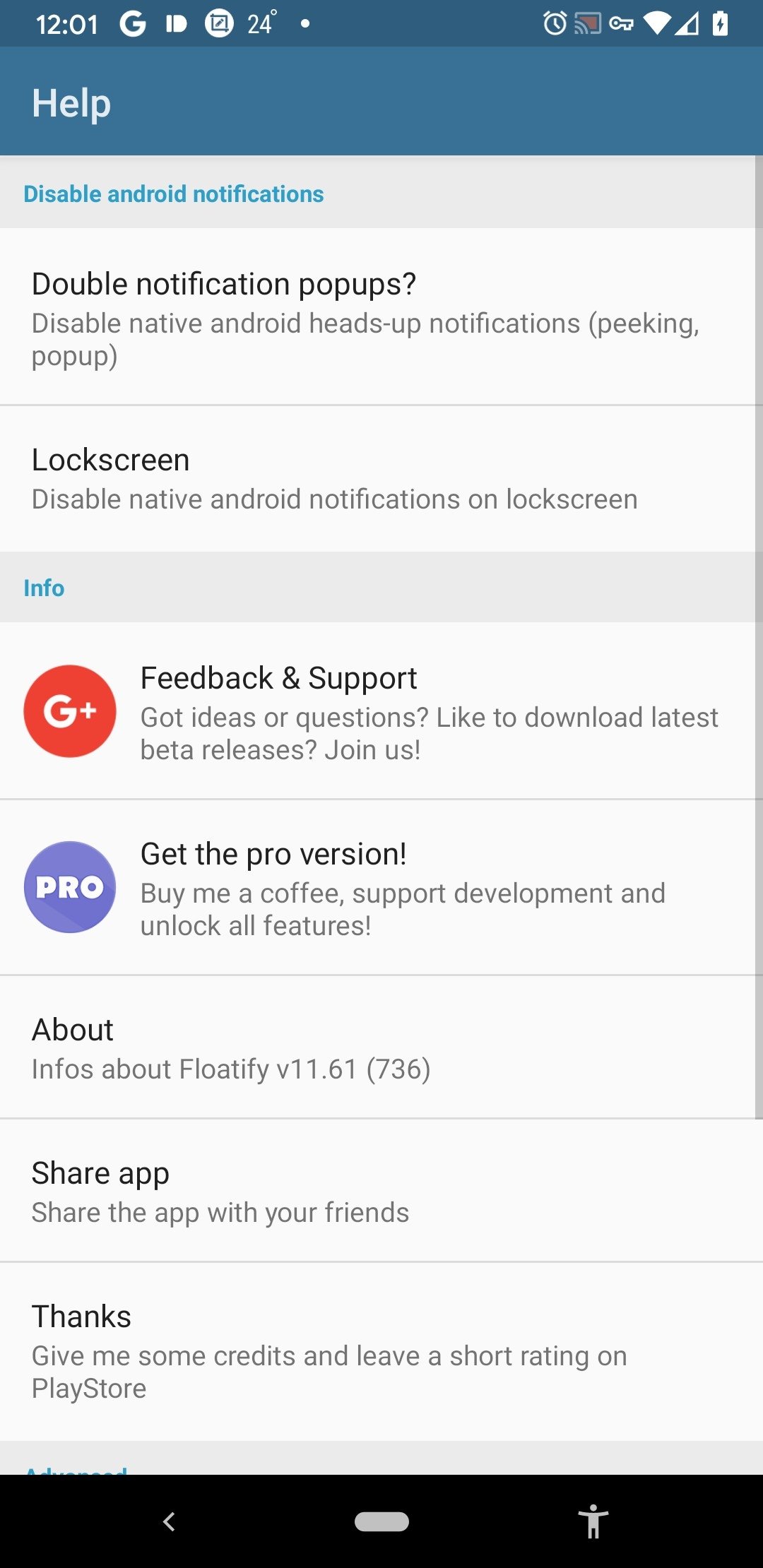**Detailed Caption:**

This image is a screenshot of a mobile application displayed in portrait mode. The interface is presented as a single long column, featuring a predominantly blue-themed background. At the very top, the status indicators show "12:01" and "24 degrees" on the upper right, next to a fully charged battery icon.

Beneath this, the background transitions to a lighter shade of blue with the word "Help" prominently displayed. Following this section, a row with a gray background contains the option "Disable Android Notifications" in blue text. The next row, set against a white background, details "Double notification pop-ups" and the option to "Disable native Android heads-up notification (peeking pop-up)."

Continuing downward, another row discusses lock screen settings, specifically the ability to "Disable native Android notifications on lock screen." A subsequent section with a gray background and blue text labeled "Info" introduces the content below.

The first row within this gray background features a red circle with a Google Plus logo inside, alongside the text "Feedback and support: Got ideas or questions? Like to download the latest betas and releases? Join us." 

Next, a blue circle containing "PRO" transitions into another note within a light purple circle encouraging users to "Get the pro version: Buy me a coffee, support development, and unlock all features."

Following this section, the "About" row introduces "Infos about Flotify (v11.6.1)." Then a "Share app" row invites users to "Share the app with your friends." The concluding row encourages users to "Give thanks: Give me some credits and leave a short rating on Play Store."

The screenshot indicates that this is the help section of an app called "Flotify," providing various informational and interactive options to the user.